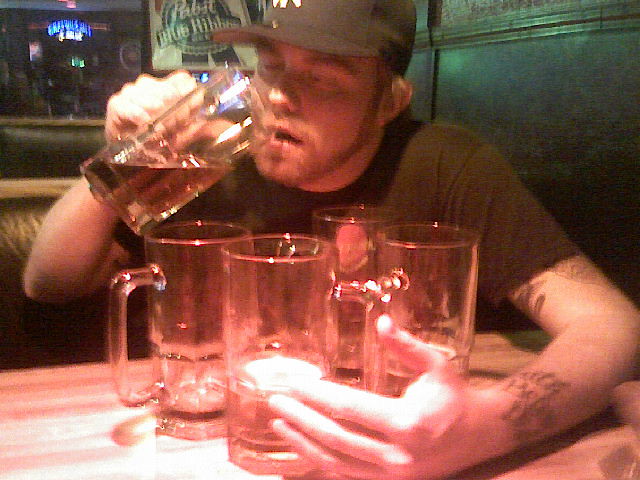In a dimly lit bar, a man sits in a cozy booth, absorbed in his drink. He wears a black baseball cap with white lettering, that closely resembles a New York Yankees cap, and a black short-sleeved T-shirt that reveals tattoos on his left arm. His left arm is affectionately curled around four empty tall beer mugs, hugging them close. He is mid-chug with his right hand holding another beer mug, more than half empty, raised to his face. His eyes are intently focused on the drink as he tilts it back. The lighting is moody, with neon bar lights, including a Pabst Blue Ribbon sign and a blue and white neon sign visible through a window, casting a colorful glow. A wooden wall behind him adds to the rustic ambiance. The man’s short, strap beard outlines his focused expression, capturing a candid moment of indulgence.